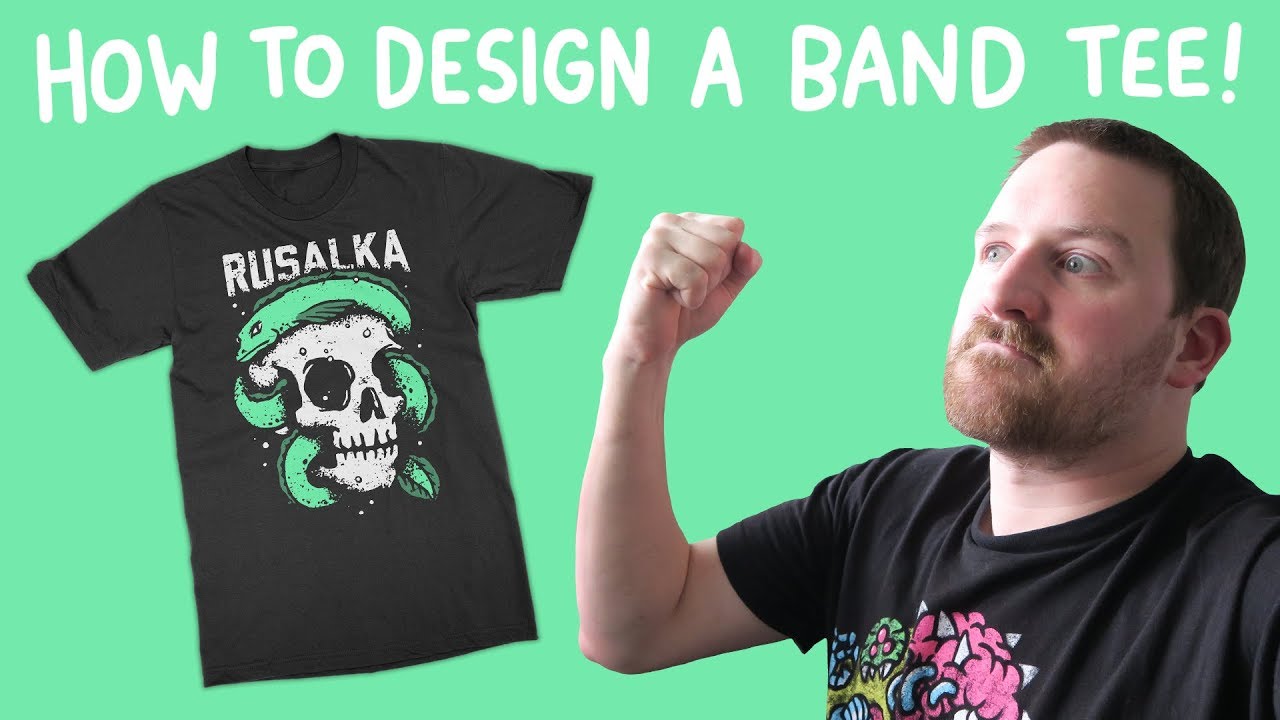The image features a YouTube thumbnail or advertisement screen on a bright light green, or mint green, background with white, capitalized comic sans text at the top that reads, "HOW TO DESIGN A BAND TEE!" On the left side of the image, there is a black t-shirt with the word "Rusalka" in white letters. Below the lettering, the t-shirt displays a graphic of a white skull with a green eel wrapping through its eye socket and jaw. On the right, a white man with short brown hair, a short beard, and a goatee mustache is shown. He has either hazel or blue eyes and a rounded ear. The man is wearing a black t-shirt, with a graphic pattern in pink and yellow, and he is holding up his right fist in an enthusiastic gesture, facing the t-shirt on the left.